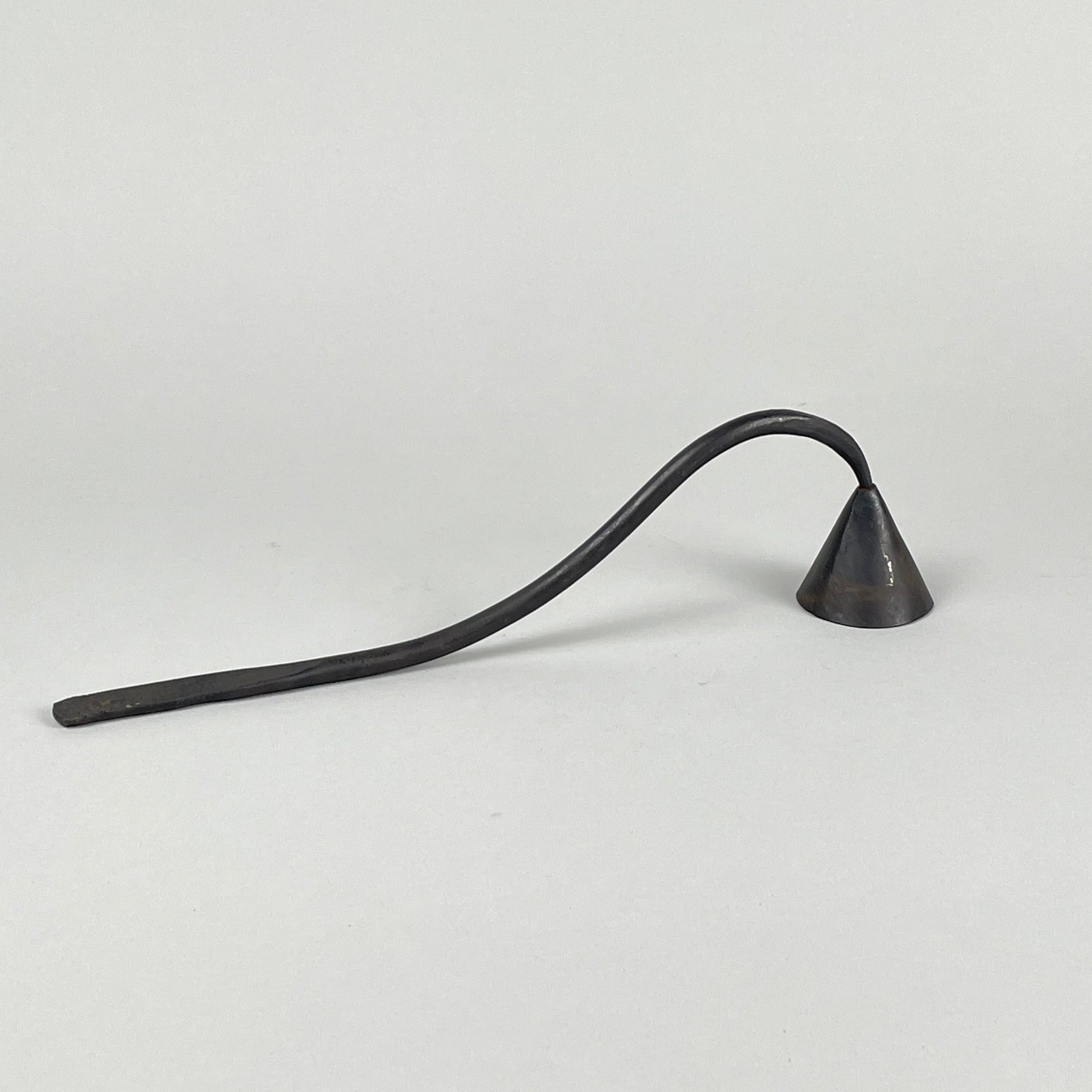This is a detailed photograph of a vintage candle snuffer captured from an angled perspective. The snuffer features a distinctive triangular cap tip with hints of tarnish or rust, imparting an aged appearance. The entire piece, including its skinny, long metal handle which curves at the top and flattens towards the bottom, is black. It resembles a miniature bell shape, akin to an upside-down ice cream cone, designed to extinguish candle flames. The snuffer is casting a shadow to the left against the plain gray background, emphasizing its dark gray coloration. The elegant curvature of the handle almost gives it a serpentine form, rising before dipping down to meet the bell-shaped snuffer cap.